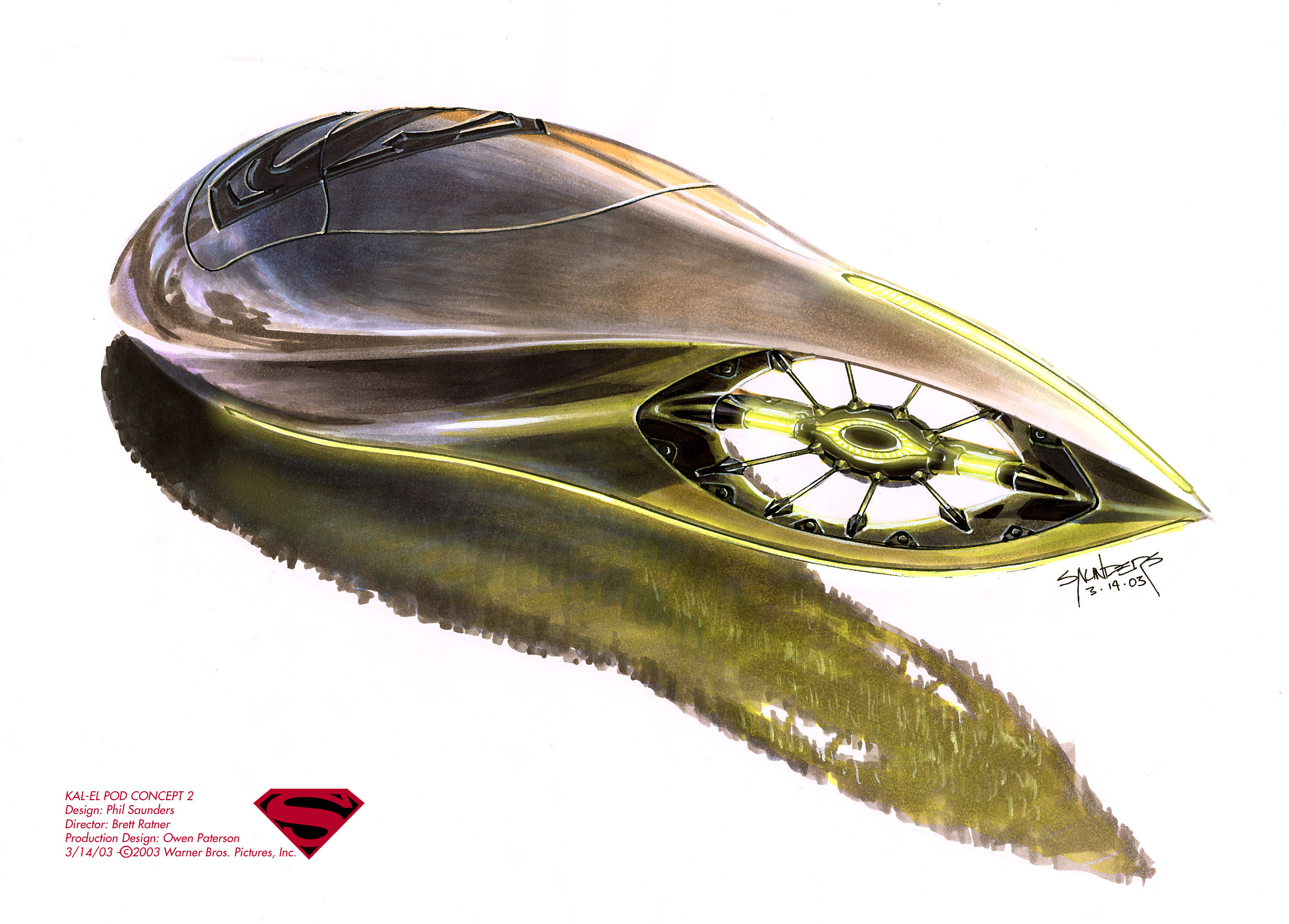The image is a detailed piece of concept art for a Superman movie, created by Phil Saunders and dated March 14, 2003. The artwork features the "Kal-El Pod Concept 2," a futuristic, aerodynamic, metallic vehicle that combines shades of grey and silver with yellow highlights towards the back. Prominent on the top is a black Superman symbol. The pod has a sleek, oblong shape with an opening on the right end and various design elements, including what appears to be a propulsion device with spikes. The vehicle's surface reflects its surroundings, giving it a mirrored appearance, possibly showing trees. The art is presented on a white backdrop, casting a shadow beneath it, and includes production details naming Brett Ratner as the director and Owen Paterson as the production designer. Saunders' signature is visible next to the thorough and alien-like design.